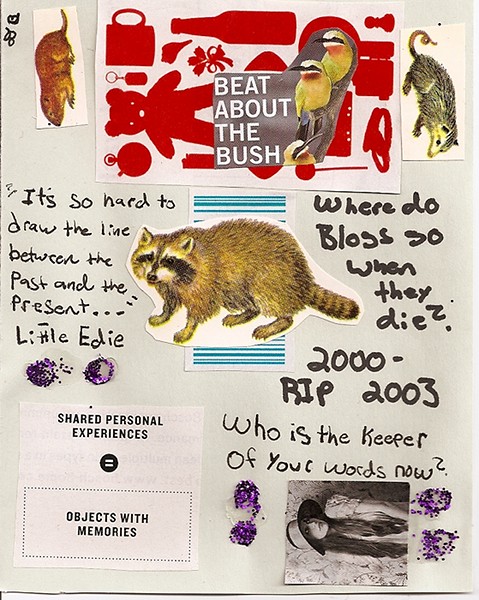The image is a detailed and intricately designed abstract art piece featuring a collage on a light grayish paper backdrop. Predominantly filled with cartoonish renderings and stickers, the composition appears somewhat scattered, resembling a school project or a journal cover. Central to this piece is a cartoon raccoon, flanked by various poignant phrases in black marker: "It's so hard to draw the line between the past and the present - Little Edie," "Where do blogs go when they die? 2002-2003, RIP," and "Who is the keeper of your words now."

Surrounding the central raccoon are several other vibrant and curious images. The top right corner showcases a sideways picture of a cartoon possum, while the top left features a similarly oriented image of a beaver. The upper middle section includes a white background adorned with red-outlined objects such as a teddy bear, a beer bottle, and a purse. Superimposed on this background is a smaller image of two yellow birds and the words "Beat about the bush" in white writing.

Towards the bottom right of the collage is a sideways image of a Caucasian woman with long black-brown hair, wearing a hat and embellished on either side with smears of purple glitter. Adjacent to this image is a white picture inscribed with "Shared personal experiences equal objects with memories" in black writing, also highlighted with purple glitter above it. Rendered in a palette of red, white, brown, purple, gray, black, yellow, and various shades of gray, the collage combines textual reflections with visual diversity, creating a piece that challenges the boundaries between the past and present.